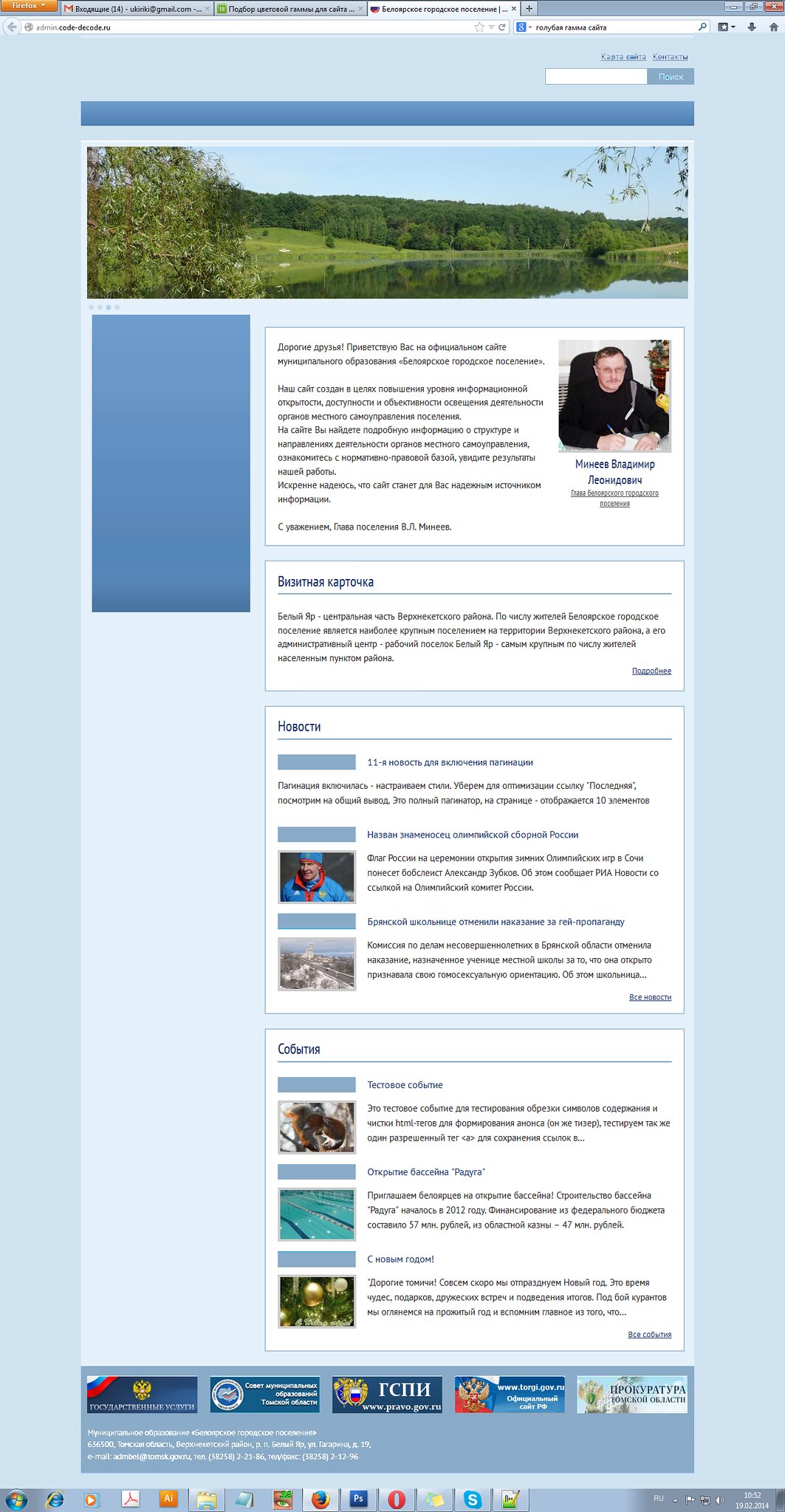The image displays a webpage in Russian, viewed on a Firefox browser. At the top, several open tabs are visible. Below the tabs, the page features a large pastoral photograph of a serene lake encircled by trees under a clear blue sky. Adjacent to this image on the right side, there's a detailed section with text in Cyrillic, likely information about a young man in glasses, dressed in black and seated on a black chair. In front of him on the desk rests a pen and some papers. Below his image and the descriptive text, the page continues with a series of smaller images and text boxes. These include photos of various individuals, a city street, and a few items such as squirrels, a swimming pool, and a close-up of a Christmas tree. Towards the bottom of the screen, advertisements are displayed alongside additional text, including mentions of specific websites like www.torgi.gov.ru. The bottom part of the page also shows several software icons, including those for Firefox, Internet Explorer, and Adobe, amidst other possible ads.